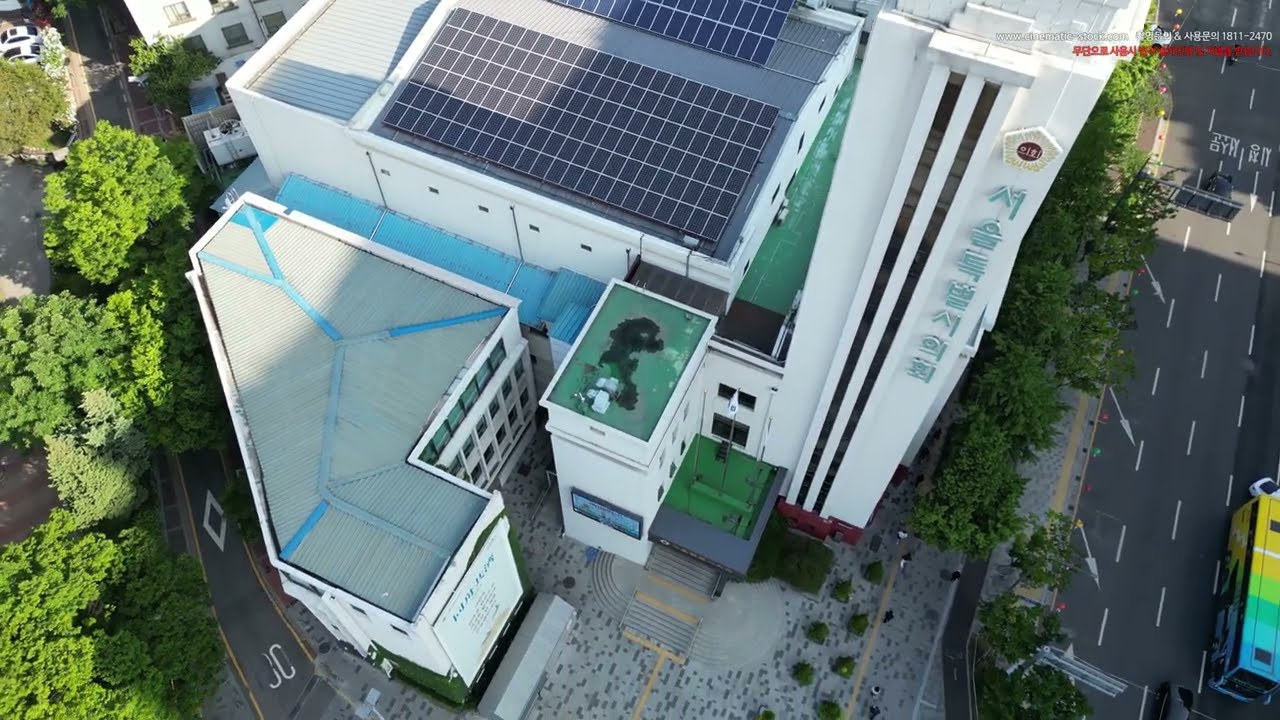This aerial color photograph, taken during the day, captures a landscape orientation view of a commercial multi-story building with a white facade. At the top of the image, the building features a large array of solar panels on its flat rooftop. Trees surround the building on the bottom left, casting a serene green backdrop. Toward the front in the bottom center of the image, there's a paved courtyard. Adjacent to the building on the right side, a multi-lane roadway runs north to south, marked by broken white lines. A multicolored bus, adorned in shades of yellow, green, turquoise, and blue, is visible in the far right lane near the bottom right corner of the image. Additionally, Chinese or Japanese characters are present on a sign vertically affixed to the building. While several people appear to be walking on the sidewalk below, it's also possible these are patches of colorful elements. In the top right corner, there is a subtle watermark with the URL "www.cinematicstock.com" in white lettering alongside text in a foreign language, with an additional line of text in red beneath it. The overall scene embodies photographic realism, effectively documenting the urban landscape with detailed clarity.